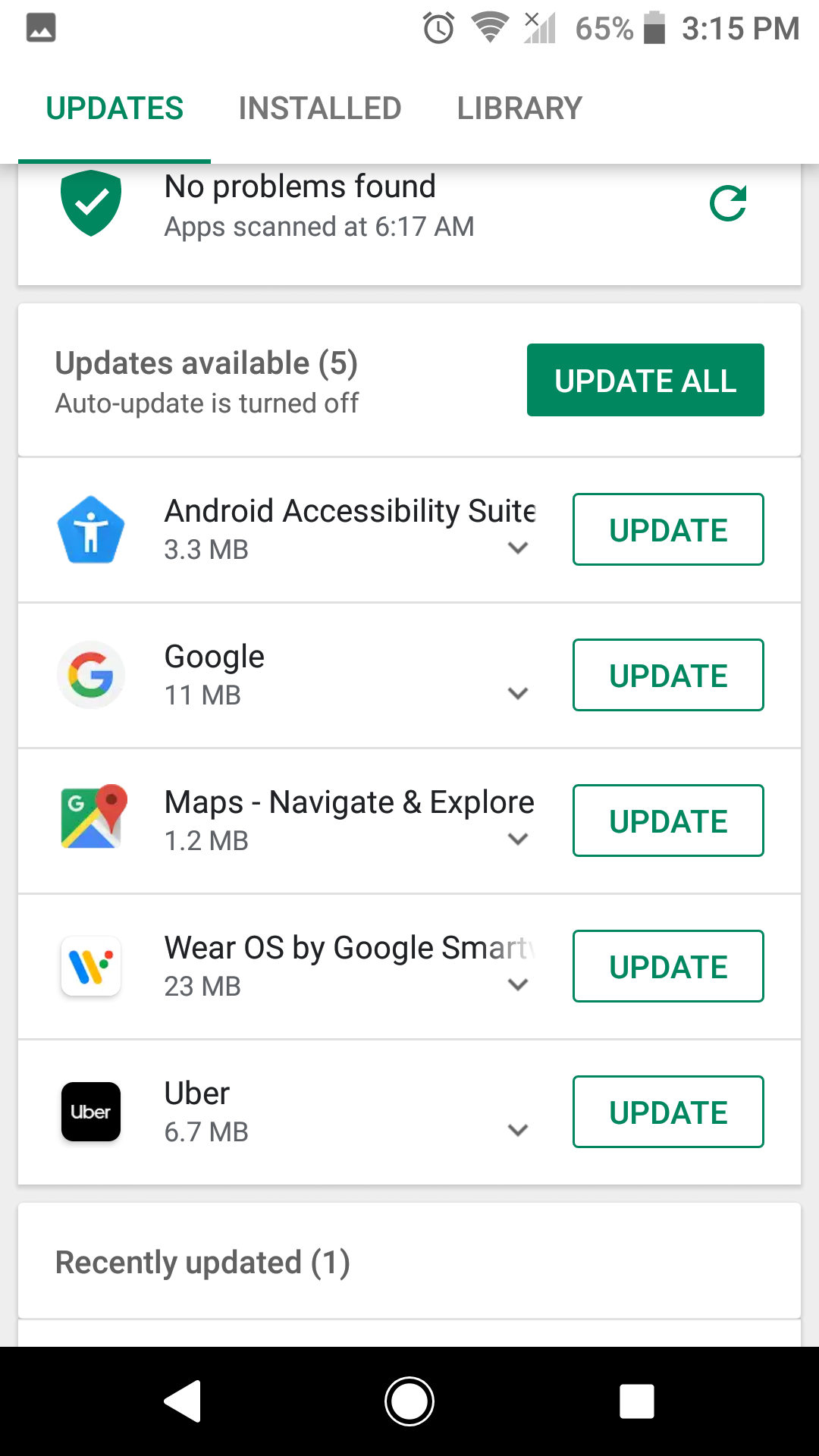This is a detailed description of a screenshot from an Android phone. At the top of the screenshot, there are standard elements visible: a profile picture, an account icon for photos, the current time (3:15 PM), Wi-Fi signal strength, and a cellular signal which is gray with an 'X', indicating no signal. The battery level is at 65%.

The screen has three tabs at the top, where the "Updates" tab is highlighted in green, while the "Installed" and "Library" tabs are in black. Just below these tabs, there is a rectangular box displaying a message: "No Problems Found, app scanned at 6:17 AM," accompanied by a circular arrow icon pointing to the right.

Further down, there's a notification stating, "Updates Available, Auto-Update is turned off, Updates Available: 5." Below this notification is a prominent green button labeled "Update All." 

Following this, a list shows the apps that require updates:
1. Android Accessibility Suite
2. Google Maps
3. Dash Navigate and Explore
4. Wear OS by Google Smart
5. Uber

Each app on this list has a corresponding button next to it with a white background, a green outline, and green text that reads "Update."